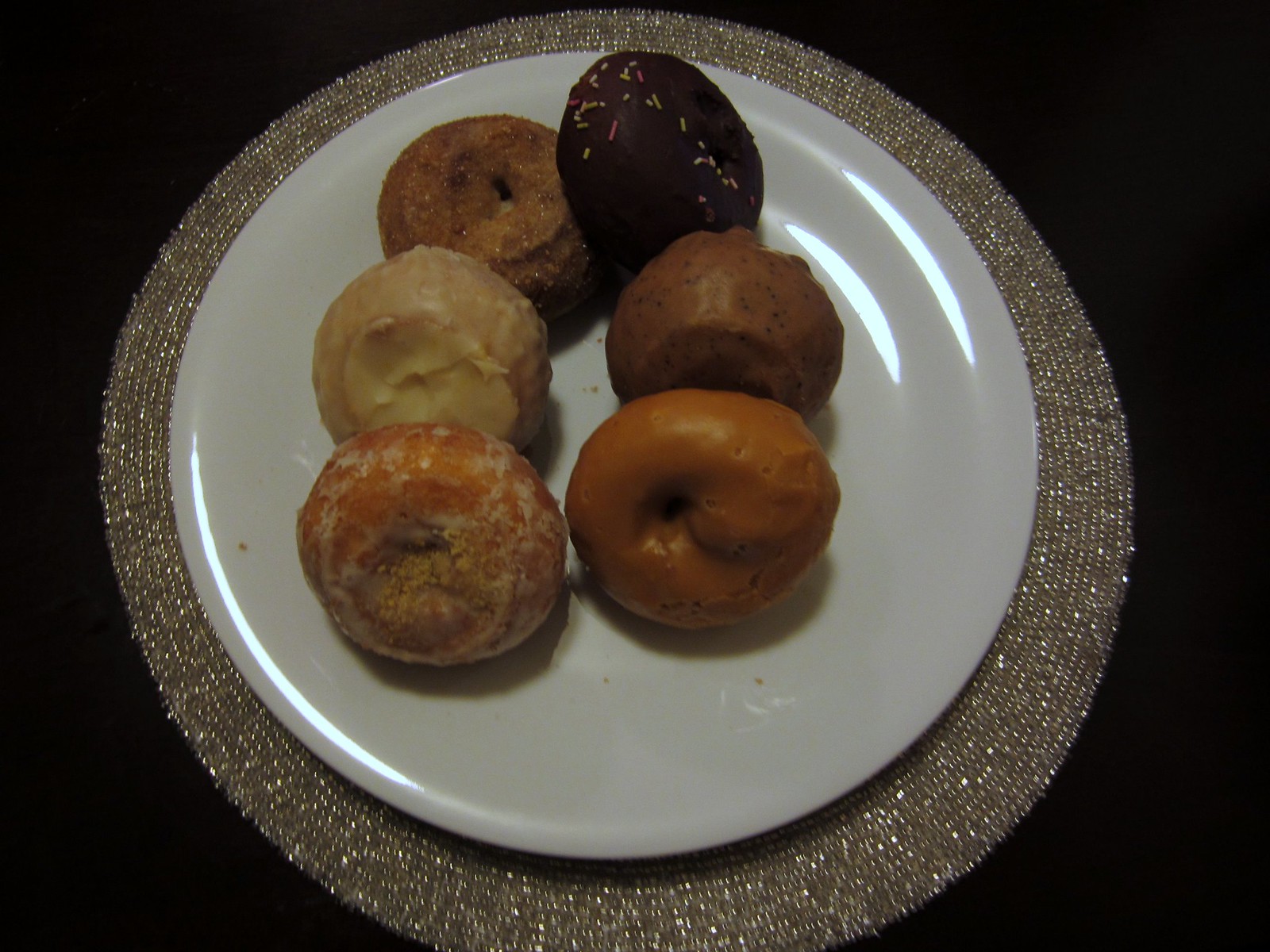A photograph features a white porcelain plate adorned with six assorted doughnuts, resting on a sparkling, silver-brown placemat. The plate, circular and glossy, is accentuated by points of light reflecting off its surface, notably at positions mimicking 2 o'clock and 8 o'clock.

The doughnuts are arranged in two loosely aligned rows. Starting from the back left, the first doughnut is chocolate-covered, adorned with colorful sprinkles. Moving forward, the next doughnut appears to have a maple glaze, and in front of that, a brown doughnut with either cinnamon or powdered sugar.

To the right, another doughnut is lightly glazed, potentially with cinnamon or vanilla, and beside it, a darker-hued doughnut, possibly caramel or molasses glazed. The final doughnut on the far right is plain yet carries a smooth, shiny finish.

The setting is further enhanced by the circular, glittery placemat beneath the plate, which gives a sophisticated contrast against the deep, dark black background, emphasizing the vibrant colors and textures of the doughnuts. The entire image, though slightly grainy and out of focus, captures a moment of inviting delicacy under a well-lit ambiance.